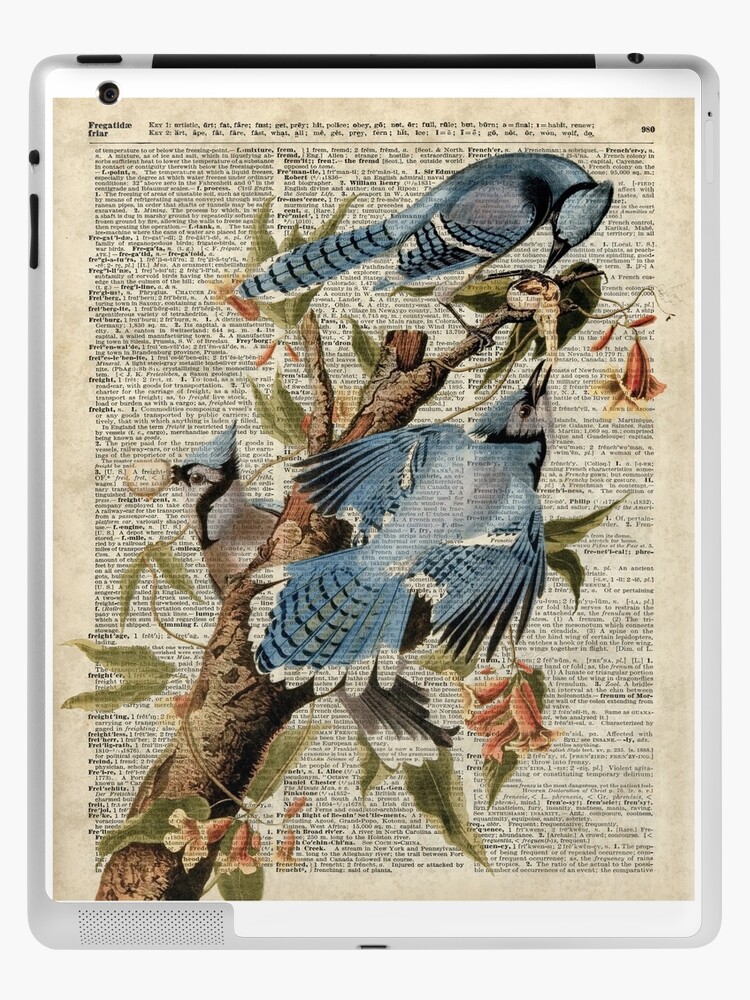The image features a dictionary page, specifically from the F section, containing the words "forget-a-day" and "friar," indicating page 980. Superimposed on this page is a vibrant painting of three blue and black birds perched on a thick tree branch with offshoots of smaller sticks adorned with green leaves and pinkish-orange, bell-shaped flowers. The top two birds, situated on the upper right of the image, appear to be squawking at each other, while the third bird, located at the lower left, looks to the left side, observing the scene. The intricate detailing of the birds and the natural elements contrasts with the text below, creating a visually striking composition.